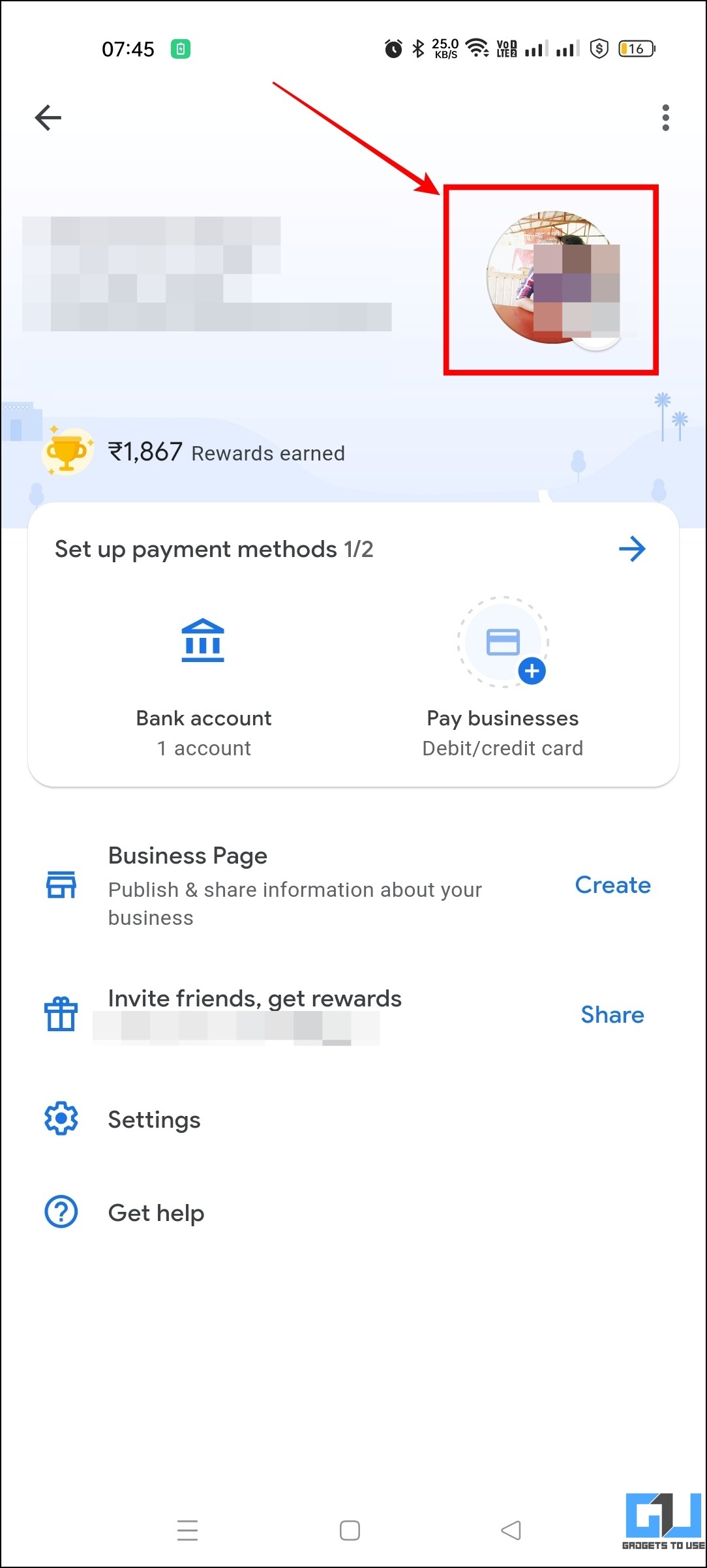This image captures a screenshot from a cell phone display, with several areas deliberately blurred out for privacy, appearing as gray and white digital blocks. At the very top of the screen, there's a back arrow icon, and the time displayed is 07:45. Immediately below, the top section's details are obscured by the blur. On the right side, what appears to be a circular profile picture is partially visible but also partially blurred. A red arrow is pointing downward from the top left area to the bottom right, drawing attention to the profile picture framed by a red rectangle.

Below this section, the content reads "Set up payment methods," followed by options such as "Bank account" and "Pay businesses." Further down, there's a partially blocked out section titled "Business page," along with options to "Invite friends" and "Get rewards," which are also blurred for privacy. Towards the bottom, the options for "Settings" and "Get help" are visible.